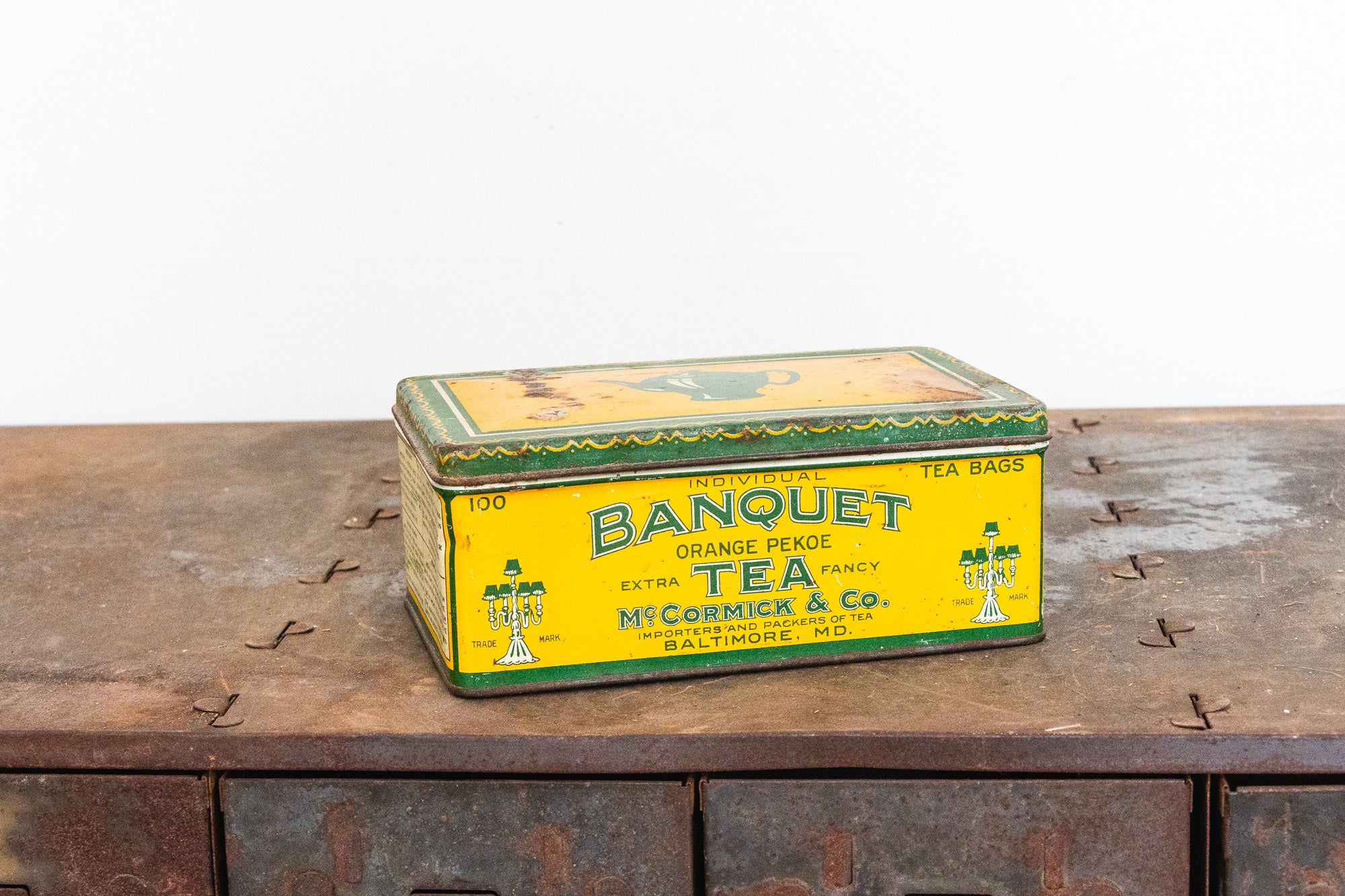This photo features a meticulously detailed vintage tin box of Banquet Orange Pekoe Tea from McCormick & Company, Baltimore, Maryland. The tin is prominently displayed atop a heavily rusted, metal table that boasts several small drawers visible at the front. The tin, approximately 8 1/2 by 6 by 4 inches in size, is a striking yellow color with green trim and blue lettering outlined in white. It is adorned with elegant floral designs reminiscent of Indian styles and features company logos that resemble lamps or chandeliers. The top section of the tin indicates it holds 100 individual teabags, with the text "100 individual teabags" arranged across its face. The lid of the tin, partially visible, displays a teapot. Despite its age and a slight hint of rust, the tin's intricate design highlights its 'Extra Fancy' nature, encapsulating a timeless charm.